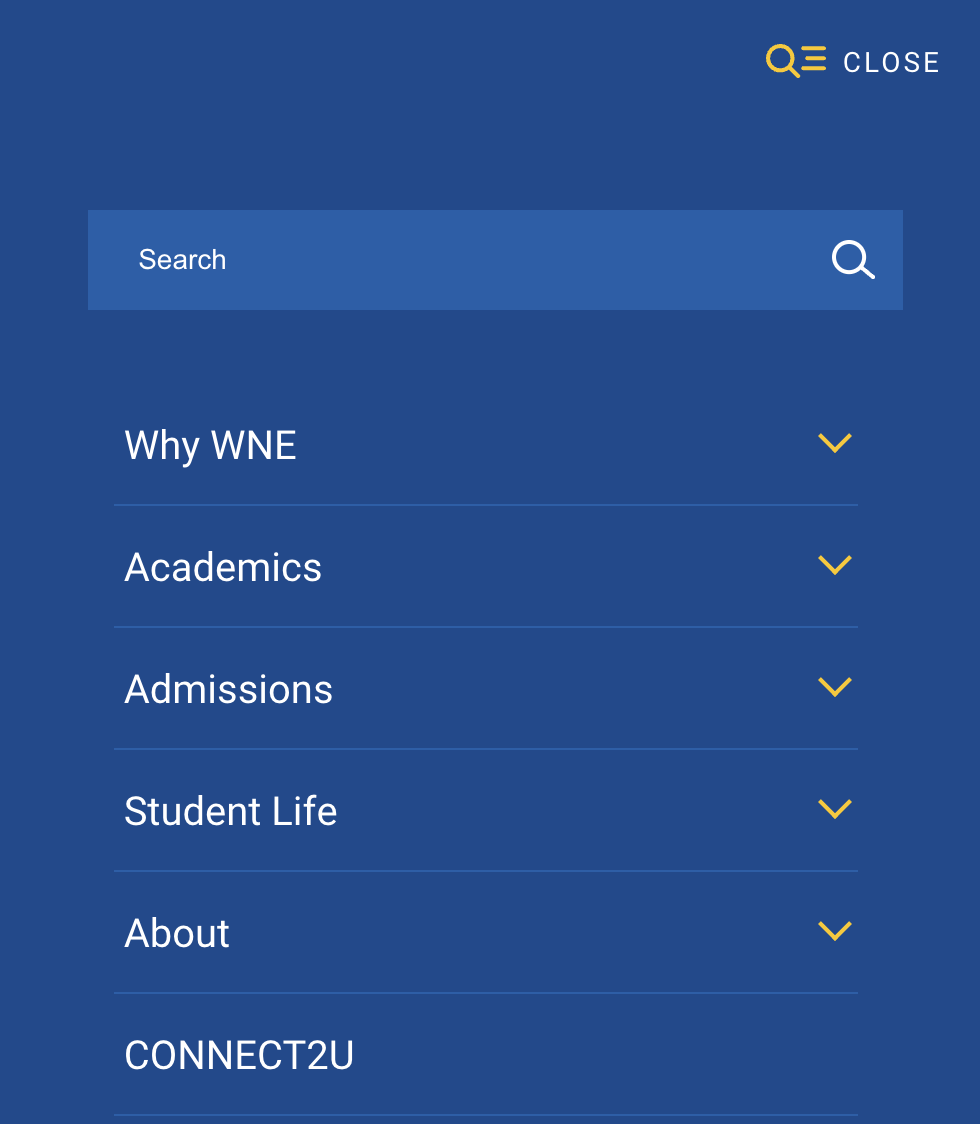The image depicts a screenshot of a college application interface on what appears to be an Android smartphone, inferred by the design of the settings icon in the upper right-hand corner. The upper right section features a yellow magnifying glass and three horizontal lines, symbolizing search functionality and settings, respectively. Adjacent to these icons, "CLOSE" is displayed in white, uppercase text, allowing users to exit the screen.

The primary color scheme of the application is navy blue, enhancing a professional and cohesive appearance. Beneath the top icons, there is a lighter blue search bar, with the word "Search" aligned to the left and an accompanying magnifying glass icon positioned to the right.

Below the search bar are multiple drop-down menu options, structured vertically. These include:

1. **YWNE** (displayed in uppercase letters)
2. **Academics**
3. **Admissions**
4. **Student Life**
5. **About**
6. **Connect to You** (also in uppercase letters)

Each of the first five options features a drop-down arrow, indicating expandable menus. The last option, "Connect to You," does not provide a drop-down menu.